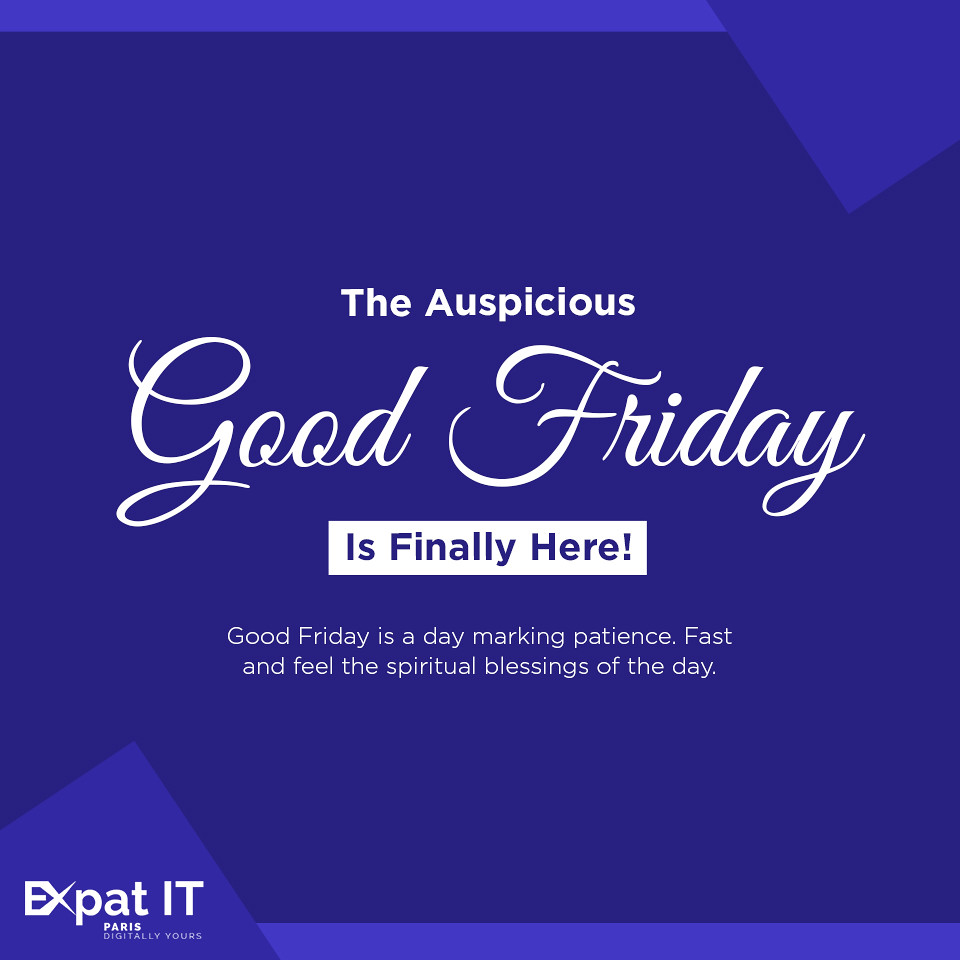The image features a predominantly blue background with varying shades of purple as accents. Centered on the design are the words "The auspicious Good Friday is finally here" in white script, with "Good Friday" presented in an italicized font. Below this, a white rectangle contains the words "is finally here" in blue letters. Beneath the central text, the caption reads, "Good Friday is a day marking patience, fast and feel the spiritual blessings of the day," also in white letters. At the bottom left, there is a logo that states "Expat IT, Paris. Digitally yours" in white. The overall design includes geometric elements, such as a light blue triangle in the upper right corner and complementary borders in lighter blue along the top and bottom of the image, further enhancing the visual appeal.